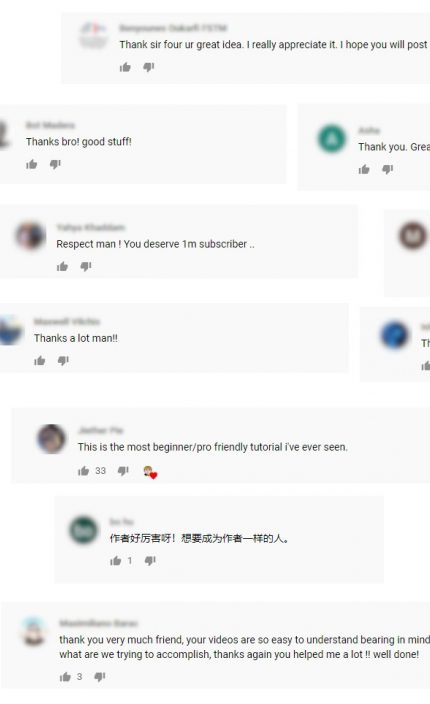This image showcases several comments on an online post, presumably on a video-sharing platform. The comments are as follows:

1. "Thanks for your great idea, I really appreciate it. I hope you will post more."
2. "Thanks bro, good stuff. Thanks, thank you, great, respect man, you deserve one million subscribers."
3. "Thanks a lot man. This is the most beginner-friendly, yet pro-level tutorial I've ever seen."
4. The fourth comment is written in Chinese.
5. "Thank you very much, friend. Your videos are easy to understand and remember. What are we trying to accomplish? Thanks again, you help me a lot. Well done."

Overall, the comments reflect high appreciation and gratitude towards the content creator for their helpful and easy-to-follow tutorials.